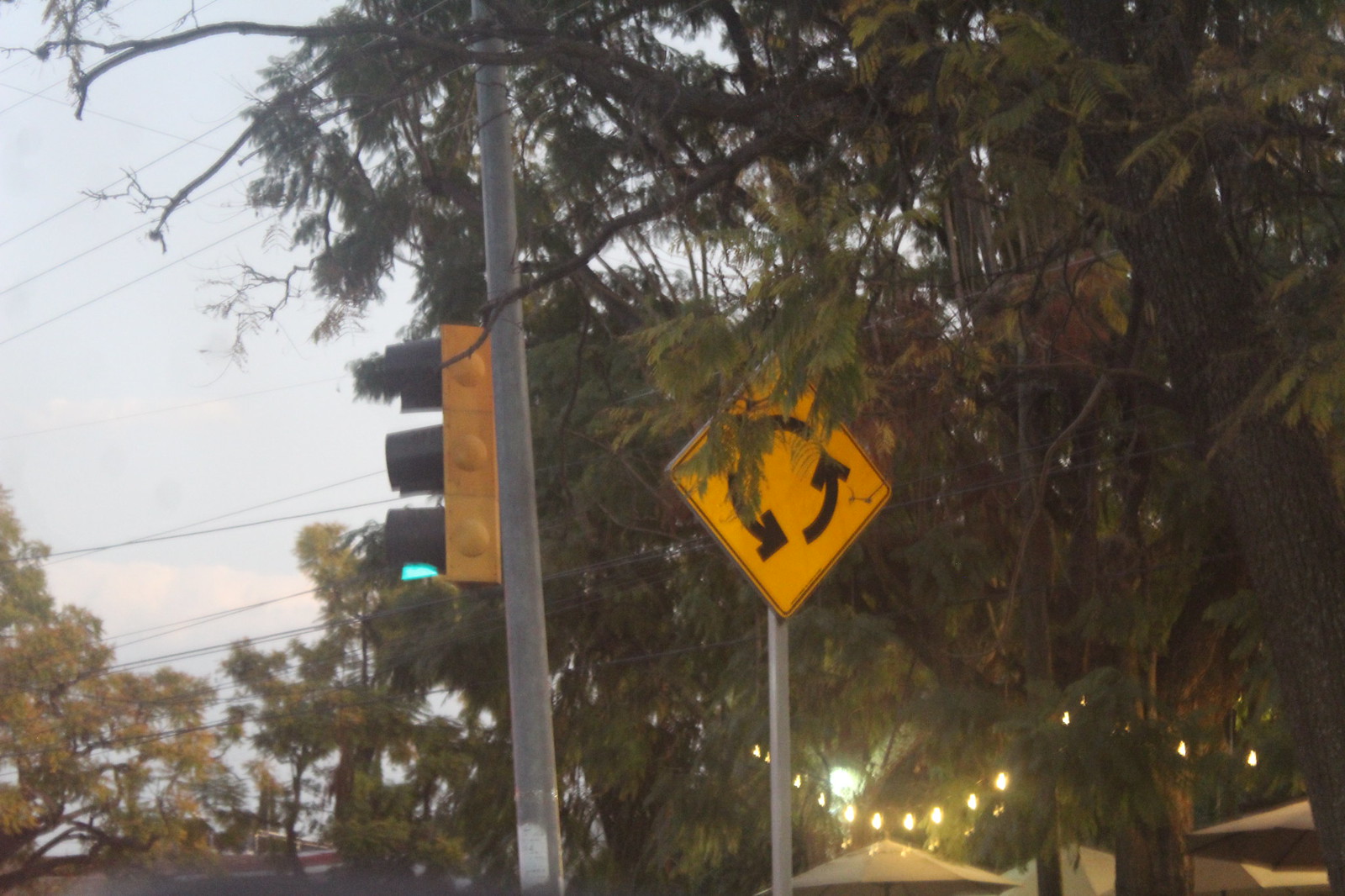This color photograph captures a bustling intersection dominated by a roundabout. Central to the image is a tall, metal utility pole, holding a yellow vertical traffic light whose green signal is just visible through its side angle. Next to it, a diamond-shaped street sign indicates the roundabout with curving black arrows. On the right, below the traffic light, are the tops of at least four white patio-style umbrellas, part of what looks like a farmers market or fair. These umbrellas are nestled among tall trees that line both sides and the background, interspersed with festive white string lights hanging above. A clear blue sky with a few clouds peeks through the dense foliage, and the scene exudes a late afternoon ambiance. The photo, slightly blurry as if taken with an older camera or in low lighting, offers a charming glimpse into a dynamic street corner framed by nature and community activities.